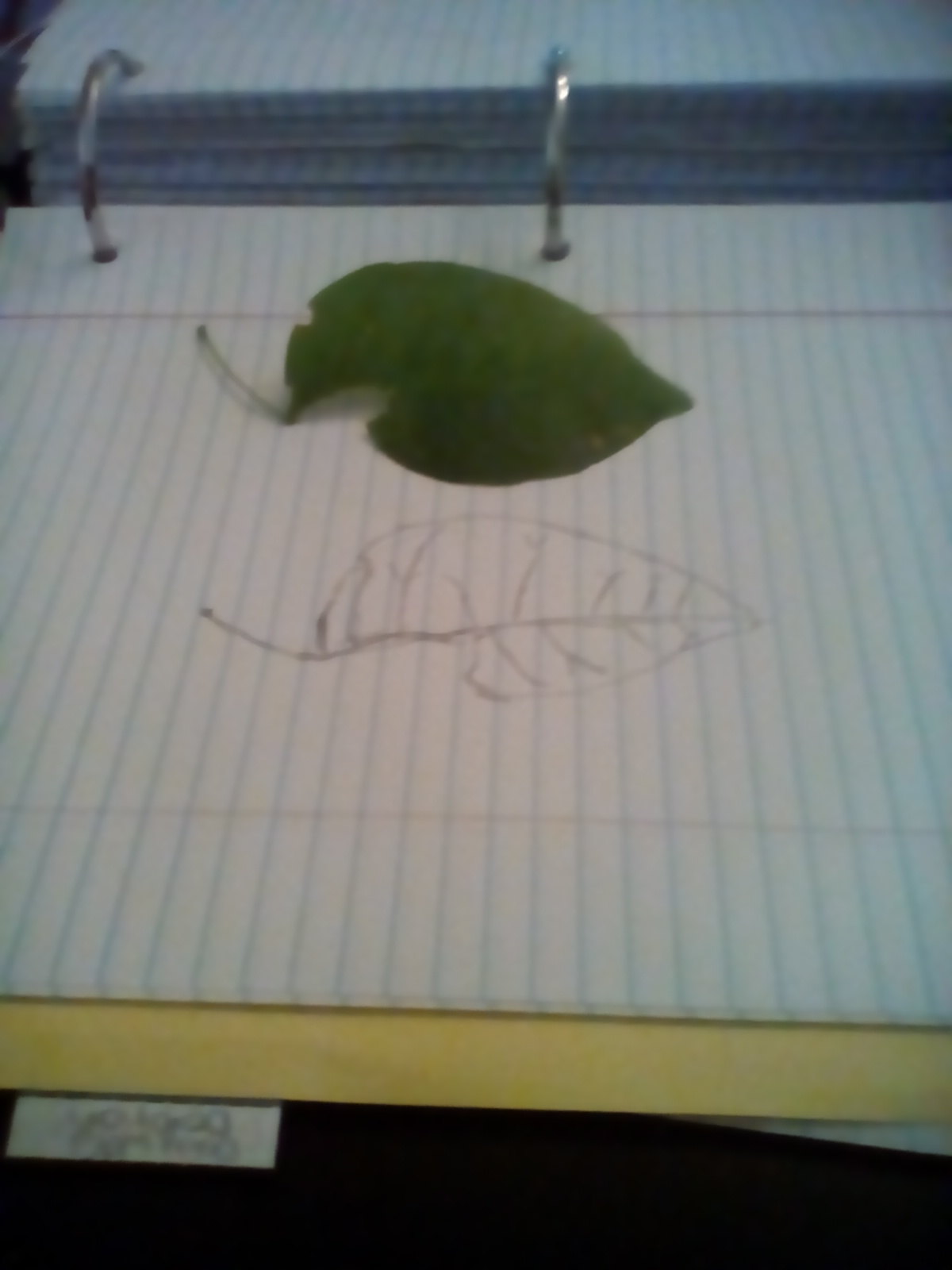In this photograph, we observe a vibrant, freshly picked green leaf resting on a sheet of white, college-ruled notebook paper. This paper, featuring a red margin line on the left, is secured within a binder, as indicated by the two visible metal rings. Directly below the real leaf, there is a meticulous hand-drawn sketch of the same leaf rendered in black ink. The artistic rendition mirrors the leaf’s structure, capturing its stem and intricate vein patterns with considerable accuracy. Positioned at the bottom of the image is a yellow divider with a white tab, albeit blurry, and some indistinct writing. The binder, filled with additional sheets of lined paper, lies on a black surface, emphasizing the main subject: the juxtaposition of the green leaf and its detailed, ink-drawn counterpart.